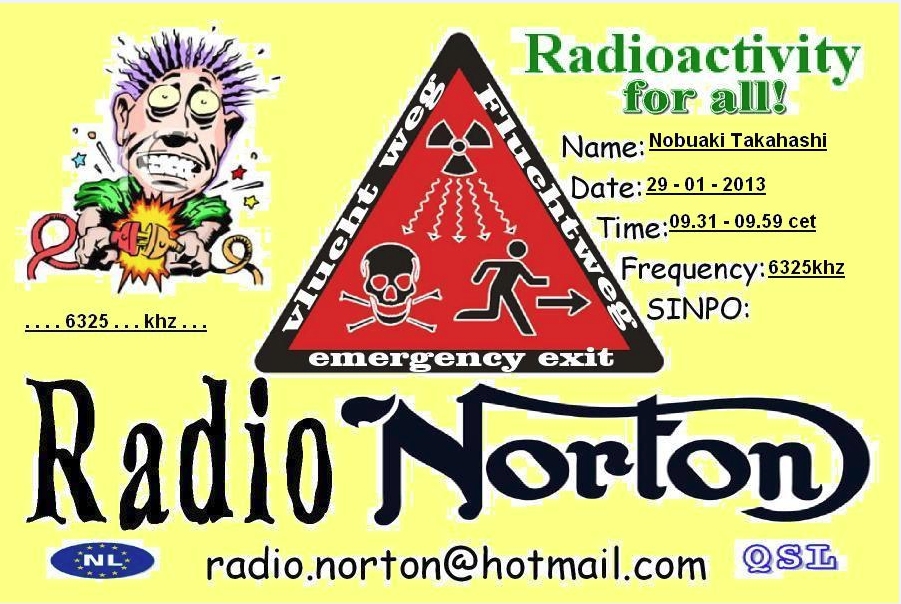This detailed poster for Radio Norton features vibrant and alarming imagery combined with important broadcast information. In the upper left corner, a cartoonish figure with frazzled hair and bulging eyes appears to be electrocuting himself by connecting two wires. He is depicted with a green and yellow body, creating a dramatic shock effect. Next to this striking image, the text "6325 KHz" is prominently displayed.

On the upper right side of the poster, in green letters, the slogan "Radioactivity for All" is prominently written. Directly beneath this, the broadcast details are listed in black text: Nabuaki Takahashi, Date: 29-01-2013, Time: 09:31-09:59 CET, Frequency: 6325 KHz, and Sensbo.

The centerpiece of the poster is a bold red triangle with a black border containing multiple alarming symbols: a radioactive warning sign, a skull and crossbones, and a figure running towards an emergency exit, emphasized by an arrow pointing to the right. The base of the triangle reads "Emergency Exit" in white lettering, while the sides feature words in what appears to be a foreign language, likely Dutch.

Beneath the triangle, "Radio Norton" is written in large, black letters against a yellow background, alongside a blue oval with the letters "NL" and elsewhere "QSL." The bottom of the poster includes the contact email "Radio.Norton@hotmail.com" in black text, flanked by the "NL" symbol and "QSL" in blue letters. The entire poster has a yellow backdrop, creating a stark contrast with the other vivid elements and further emphasizing the urgency and energy of the broadcast advertisement.